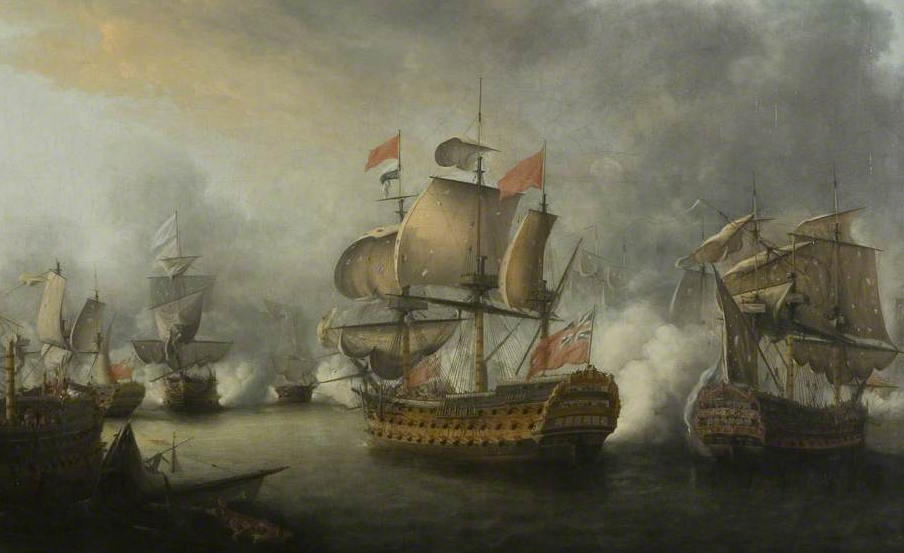Title: "Naval Battle Amidst Smoky Skies"

Description: This detailed and atmospheric oil-on-canvas painting captures an intense naval battle scene from the 19th century. The square, borderless image showcases multiple wooden sailing ships engaged in combat on a still, dark, brownish sea. The scene is dominated by a smoky, cloud-covered sky, adding to the dramatic tension of the confrontation.

Central to the painting is a prominent warship featuring a partially recognizable flag that combines the Union Jack with a red field, suggestive of a historical British naval vessel. This central ship, equipped with numerous cannons and relatively intact sails, contrasts with another vessel to the far right, which is riddled with cannonball holes.

Additional ships populate the left side of the scene, their positions partially obscured by clouds of smoke from the continuous cannon fire. The ships all have their sails fully extended and move in a coordinated fashion, possibly indicating a fleet departing from or defending a port. Vibrant flags—red, blue, and some with possible white or beige banners—flutter atop the masts, denoting various affiliations and adding splashes of color to the otherwise muted palette of browns and grays.

Overall, the painting evokes the chaos and grandeur of a maritime war, with its dark and foreboding sky, detailed rendering of the ships, and the palpable sense of smoke and fire enveloping the scene.